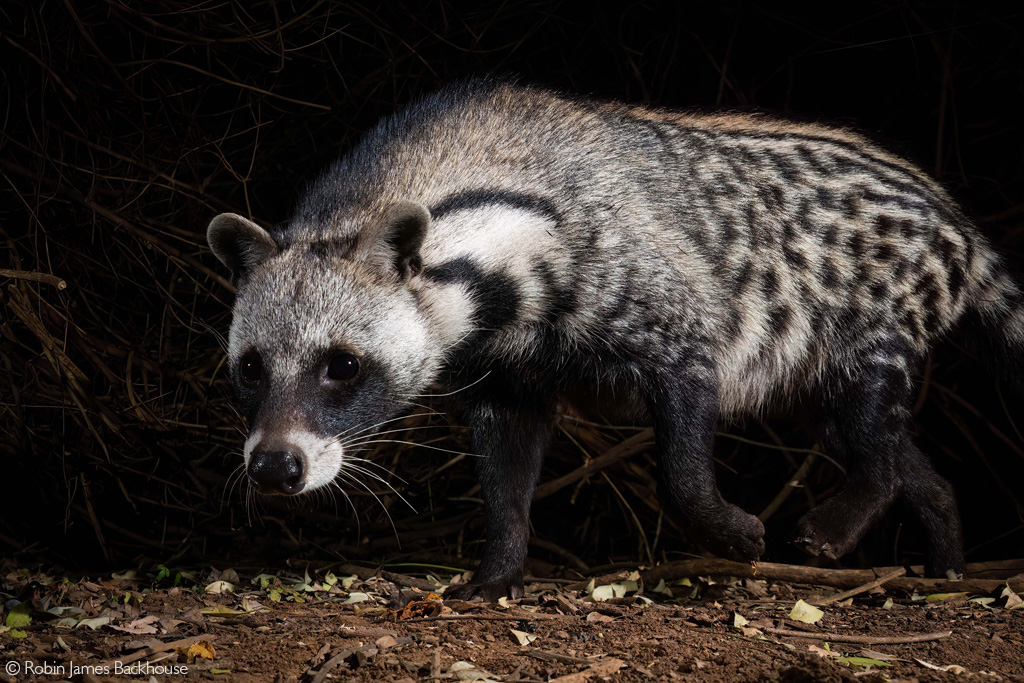The photograph depicts an unusual small animal that resembles both a raccoon and a hyena but is difficult to precisely identify. The animal, captured in a wide vertical rectangular image, is seen in a side view facing to the left, standing on all fours with its head and neck close to the ground, amidst a natural, outdoor setting. Its fur coat is predominantly gray, with the back half displaying distinctive gray spots and a hint of brown. The animal's face features striking black markings around the eyes, with a white area around its black nose. Both its front and back legs are black from the bend downward. Additionally, its neck is almost white with visible black stripes. The image appears to have been taken at night, indicated by the black sky backdrop and the dimly visible surroundings, which include brown dirt, scattered twigs, leaves, small green plants, and possibly some small pebbles. At the bottom left of the photograph, in white font, the name "Robin James Backhouse" can be seen.